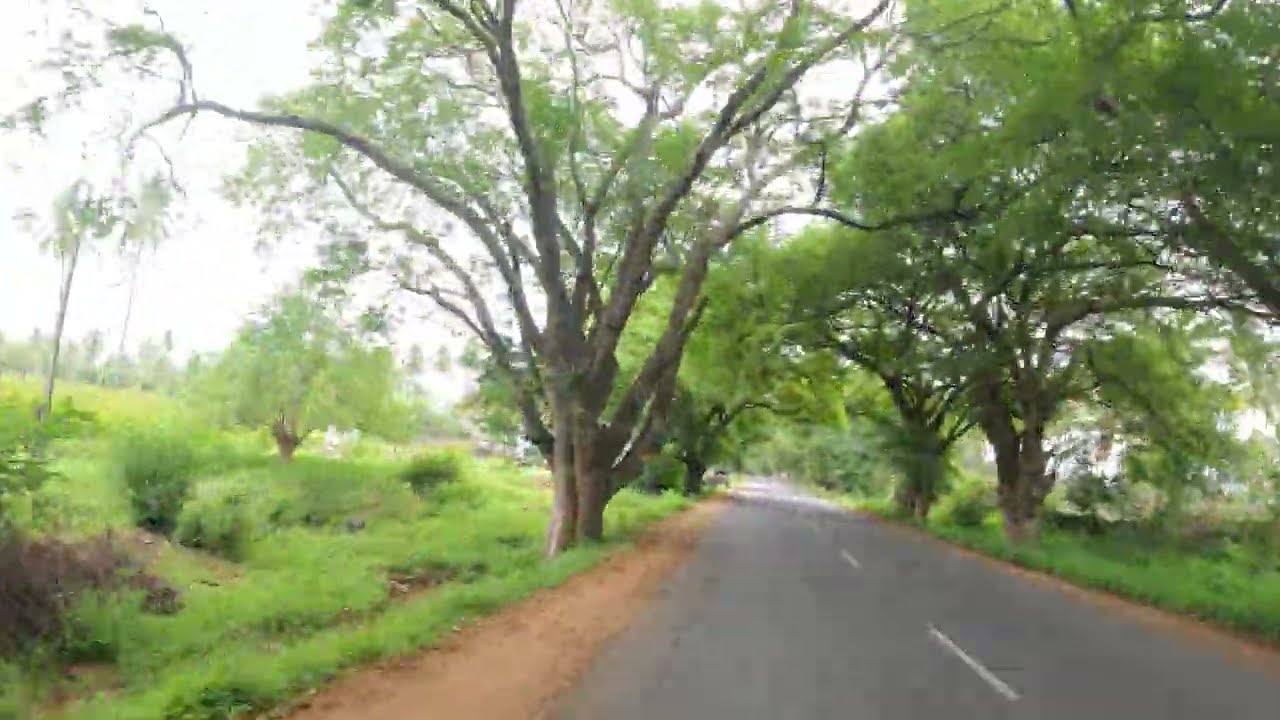This horizontally aligned, somewhat blurry image captures a serene, rural scene dominated by a narrow, two-lane paved road marked with white dashed lines down the center. The road, curving slightly to the left, extends from the bottom of the frame towards the upper left-hand side, intersecting a natural landscape devoid of buildings or people. On either side of the road, strips of flat dirt shoulder transition into areas of tall, green grass that blend into an expansive, overgrown field. Thick groves of trees with lush green leaves densely border both sides, with two prominent trees on the right and a notable large tree near the center-left of the image. The scene is completed with an expanse of white sky visible through the tree branches, bathing the area in a bright, natural light. The overall palette of the picture includes the grays of the road, the browns and blacks of tree trunks, and varied greens of the grass and foliage, contributing to a calm, isolated, and quintessentially rural atmosphere.